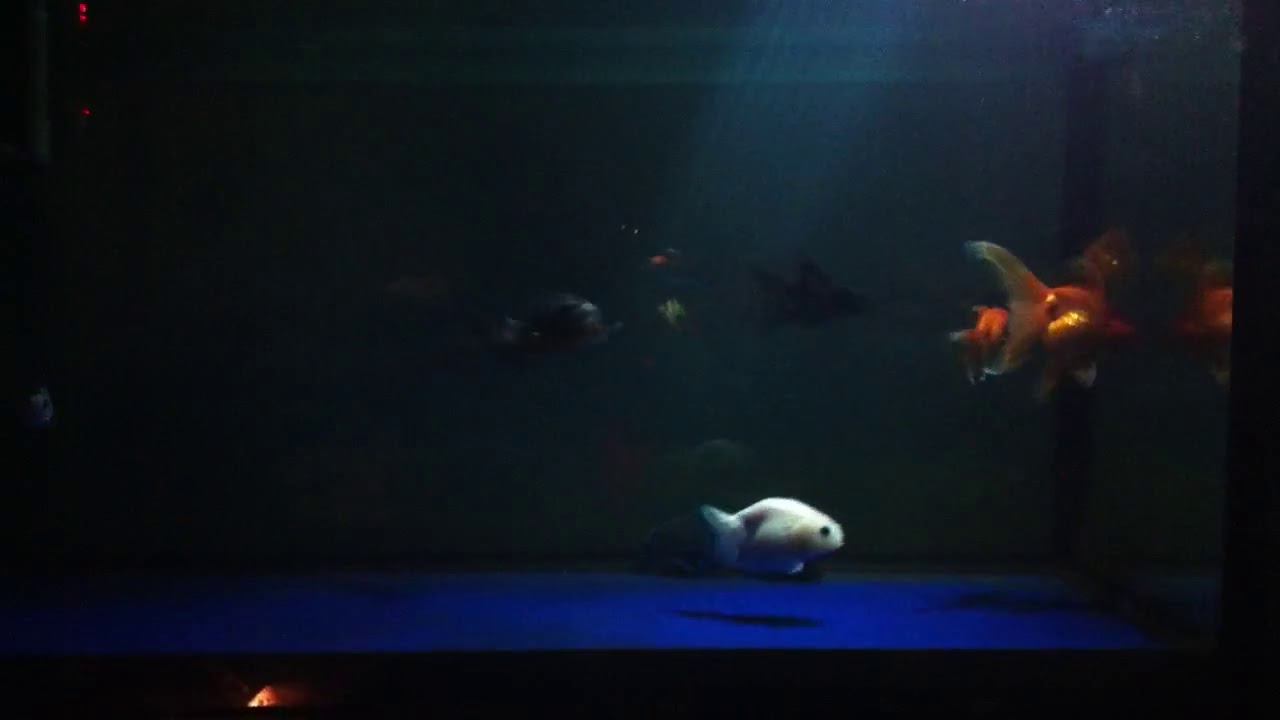The image depicts a sizable fish tank with a somewhat dim and murky atmosphere, contrasted by a blue light illuminating the water. It showcases a variety of fish, including one white fish, two black fish, and two orange or gold fish. The gold fish are positioned on the right side of the image, while the black fish are more centrally located and slightly towards the background. The white fish is closer to the foreground. The blue light reveals the tank's blue bottom, casting shadows of the swimming fish. The fish appear to be aimlessly swimming in different directions within their spacious enclosure, likely awaiting food. The overall scene is dark, with most of the light concentrated on the fish, enhancing their visibility against the otherwise shadowy environment.